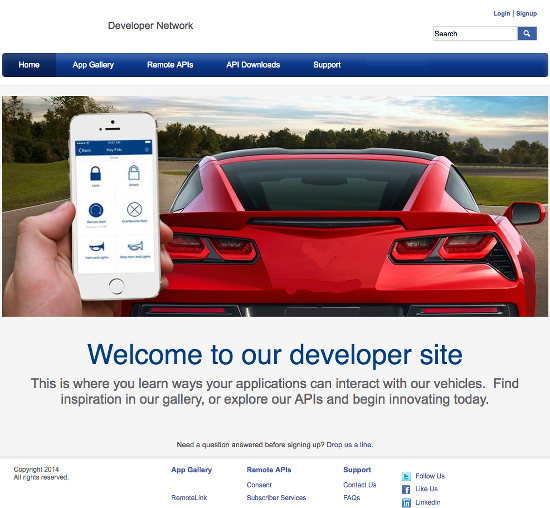Screenshot of a Developer Network Webpage

The screenshot captures a web page from a developer network. At the top of the page, a header in gray text reads "Developer Network." Positioned in the upper right-hand corner is a search bar. Just above this search bar, two links are labeled "Log In" and "Sign Up."

Below this section is a blue toolbar featuring white text headers that read: "Home," "App Gallery," "Remote APIs," "API Downloads," and "Support." 

Following the toolbar, the hero section displays a striking image of a sports car on a lush, green road. Surrounding the road is a verdant field with trees visible in the background, set against a sky with blue hues and scattered white clouds. The bottom-left corner of this image showcases a hand holding an iPhone, displaying some app icons.

Beneath the image, a welcoming message in blue text reads, "Welcome." The background here is gray, and the accompanying text elaborates, "Welcome to our developer site. This is where you can learn ways your application can interact with our vehicles. Find inspiration in our gallery, or explore our APIs and begin innovating today." This final section of text appears in gray.